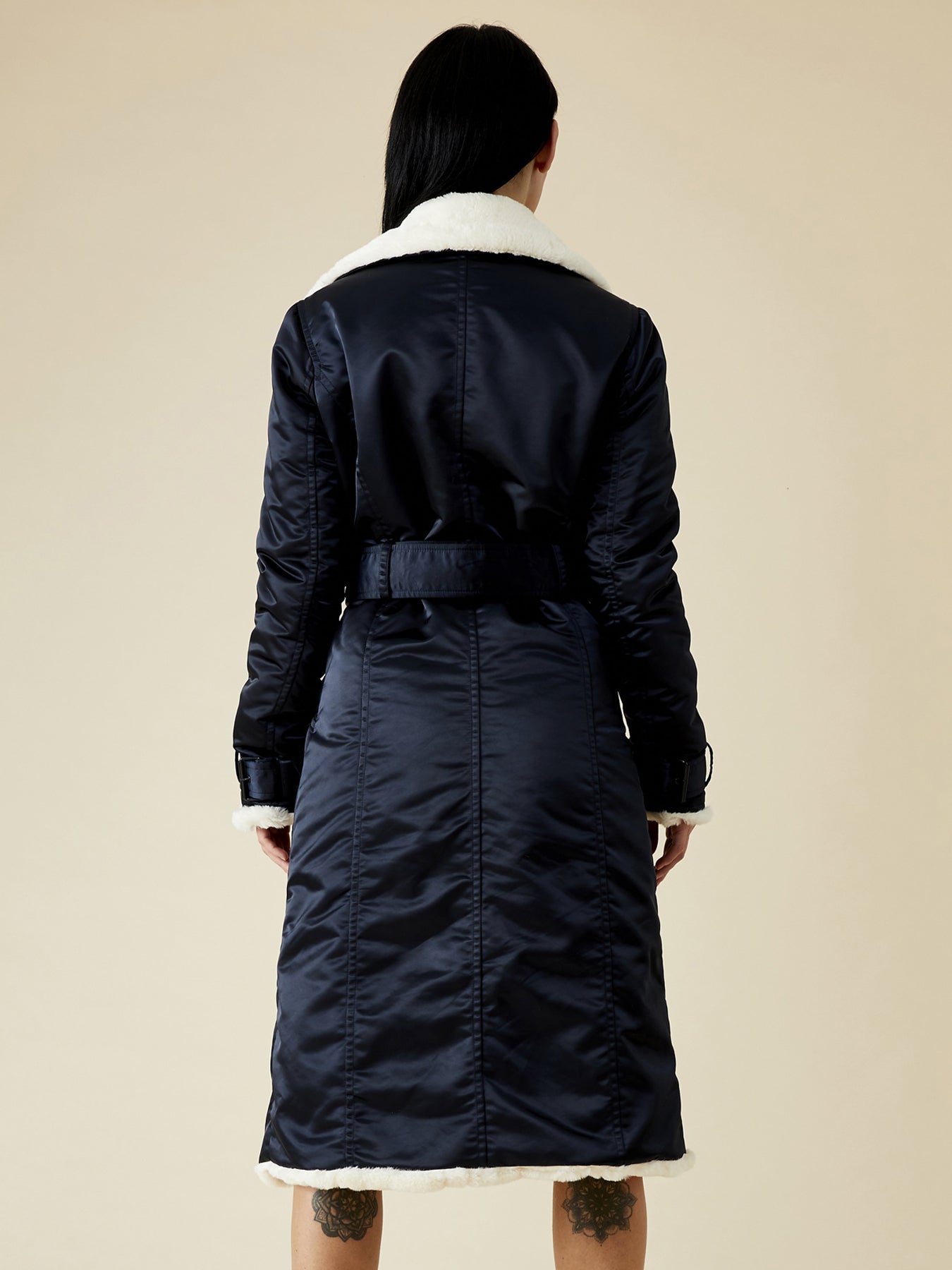This color photograph captures a striking woman standing with her back to the camera, positioned against a plain beige background. She dons a sophisticated black jacket, which may be crafted from leather or vinyl, extending to just below her knees. The jacket is adorned with elegant white fur-like trim at the collar, sleeve ends, and hem, adding a touch of luxury. A black belt cinches her waist, enhancing the jacket's structured silhouette. Her long, black hair cascades forward over her left shoulder, revealing her right ear. Her arms hang relaxed at her sides as she looks straight ahead. Intriguing tattoos, resembling symmetrical floral mandalas, adorn her visible calves, adding an element of personal expression to her fashionable ensemble.